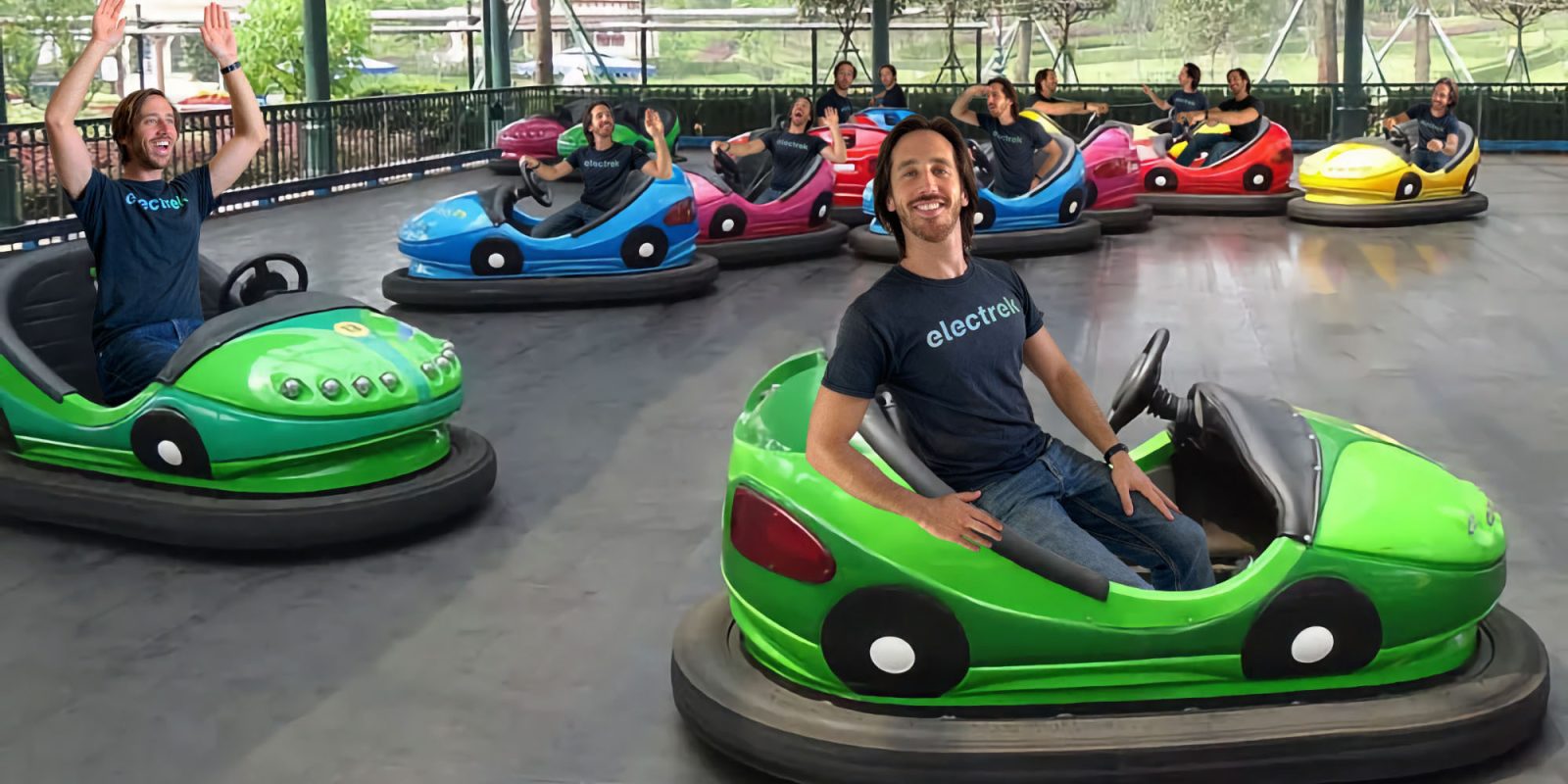This digitally manipulated image showcases a lively bumper car scene at an amusement park, featuring the same man seated in each of the numerous bumper cars. The assorted cars are vividly colored in greens, blues, pinks, reds, and yellows, contributing to the vibrant, Dayglo aesthetic of the ride. Prominently, two green cars are positioned at the front, with the man sitting calmly in one and raising his arms in another, suggesting various states of engagement and enjoyment. Sporting a black T-shirt that reads "electruck" in light blue lettering, the man with longer black hair and black stubble appears repeatedly throughout the scene. The backdrop reveals a gray cement raceway bordered by a railing, with distant hints of a golf course and trees visible through windows, indicating the park setting. This image, likely created for advertising purposes, creatively captures the dynamic atmosphere of a traditional amusement park bumper car ride.